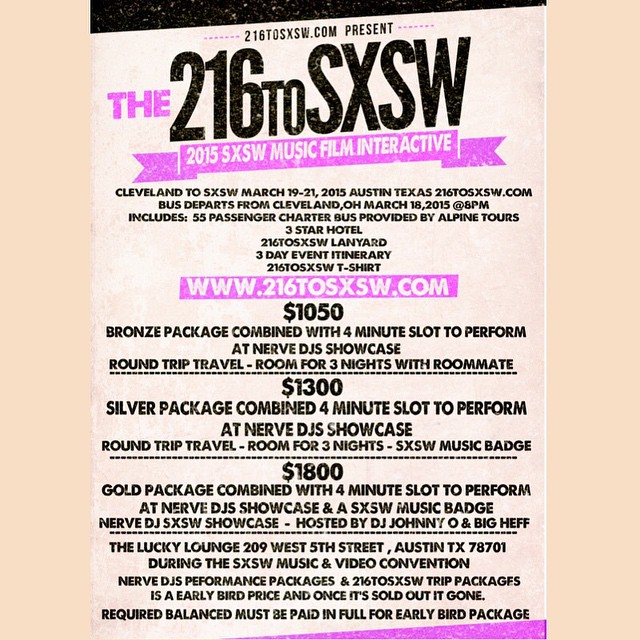The flyer advertises the "216 to SXSW 2015" event, combining music, film, and interactive experiences at the South by Southwest (SXSW) festival. The top section features the headline "216 to SXSW.com presents the 216 to SXSW 2015 SXSW Music, Film, Interactive," along with a brief schedule of the event, from March 19th to 21st, 2015, in Austin, Texas. It outlines three package tiers: the Bronze Package for $1,050, the Silver Package for $1,300, and the Gold Package for $1,800. Each package includes a four-minute performance slot at the Nerve DJs Showcase, round-trip travel, and three nights of accommodation with roommates. The flyer also provides detailed location information, specifying the Lucky Lounge at 209 West 5th Street, Austin, Texas, as the venue. There is a note that the early bird prices require full payment, emphasizing the limited availability. The flyer is designed on a tan paper background.